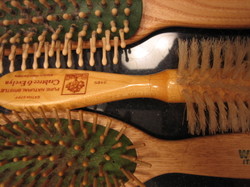This is a close-up, square-cropped photo taken from above, depicting three hair brushes with wooden handles. The brushes on the top and bottom are identical, featuring oval shapes and green pads holding numerous large, pointy wooden bristles that facilitate deep brushing. Both of these brushes, facing left, also have some green writing on their edges. The middle brush stands out with its glossier finish, red writing (illegible due to the small image size and positioning), and three rows of white bristles resembling a toilet bowl cleaner. This brush appears to have natural bristles made of some sort of animal fur or fiber, contrasting with the synthetic appearance of the top and bottom brushes.